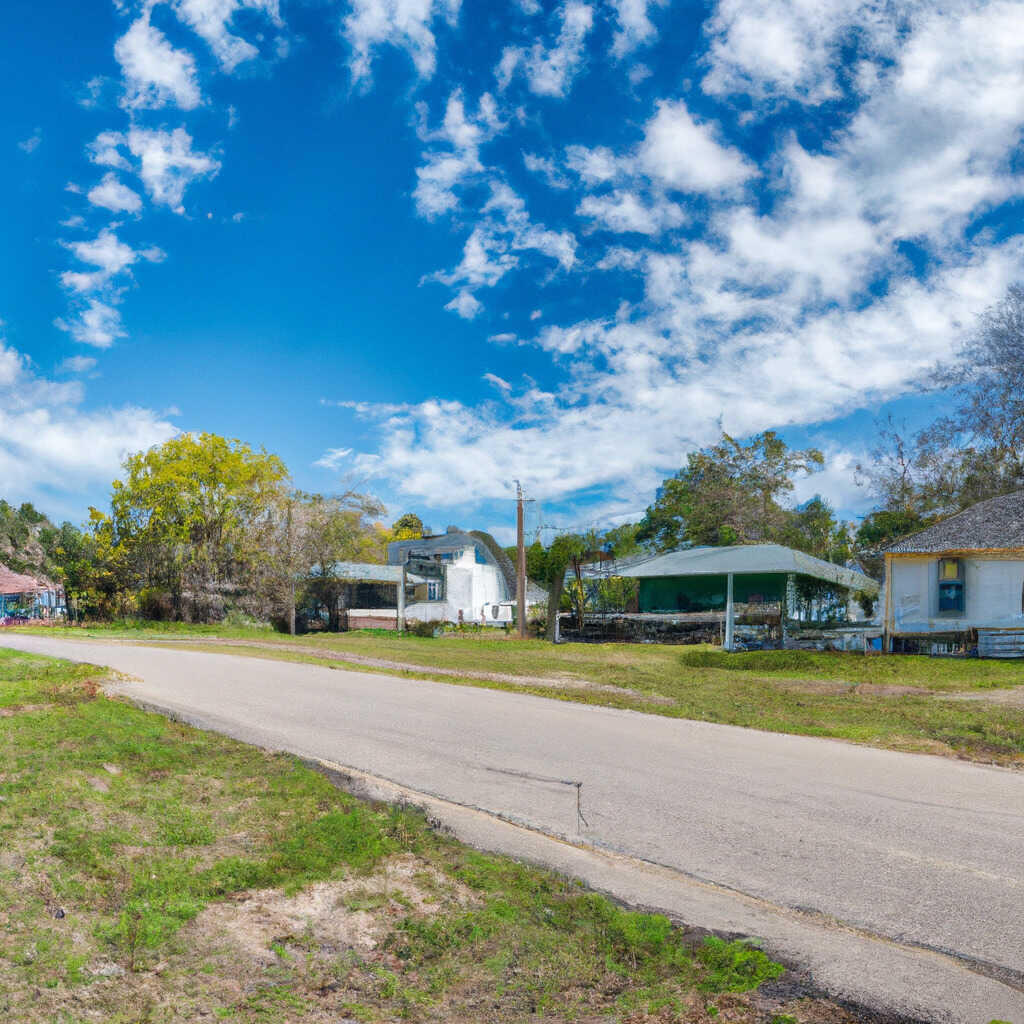This photograph captures a quaint and cozy countryside neighborhood taken during the daytime. Centered in the image is an old concrete road stretching down the street, edged by sparse bits of grass and dirt pathways on both sides. The road appears light gray and narrows as it approaches the middle of the frame. On either side of the street are small, possibly single-family houses that seem aged, contributing to the nostalgic feel of the scene. These homes, likely two-bedroom, one-bathroom types, are positioned closely together, creating an intimate neighborhood atmosphere. Surrounding the houses are a mix of trees and power lines, adding to the rustic charm. A sprawling sky overhead, occupying about half of the image, is painted a bright royal blue adorned with long, white clouds, enhancing the picturesque and serene quality of the setting. The clear, stunning sky elevates the beauty of this small town, making it appear more idyllic and inviting.